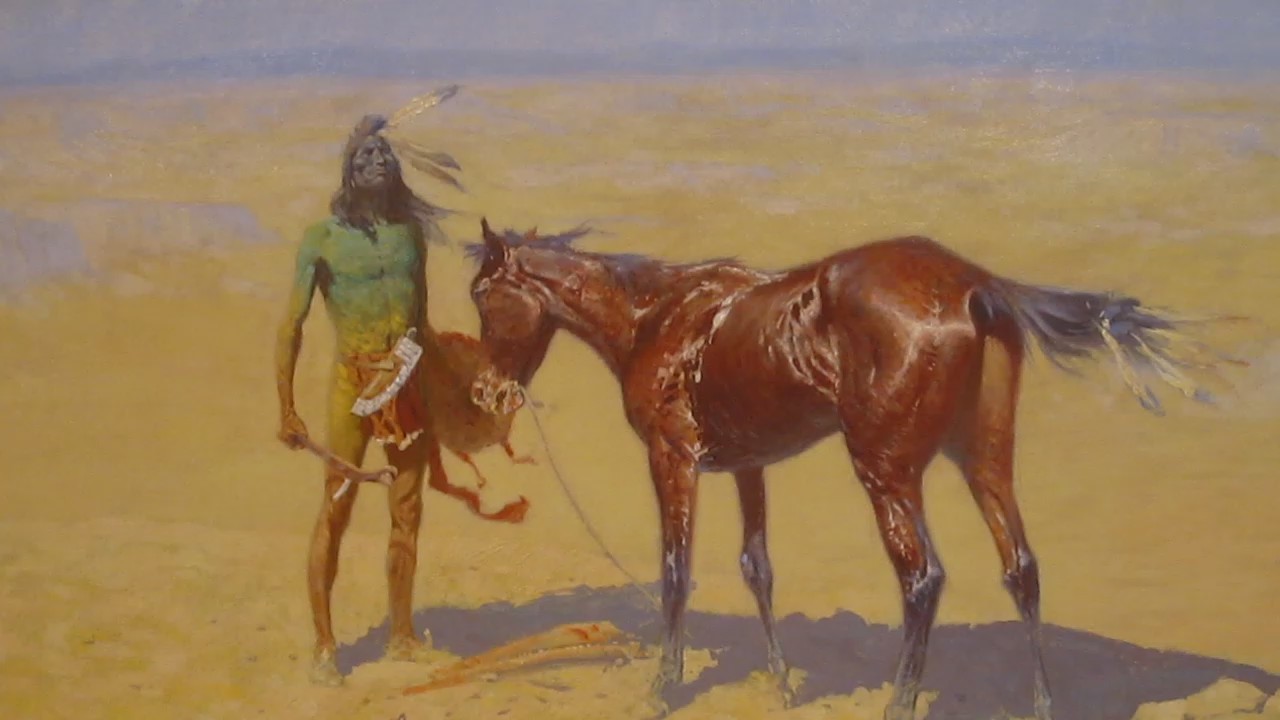The detailed oil painting depicts a Native American man standing in a desolate, desert-like environment, resembling the landscapes of Arizona or Utah, with sand covering the ground and a distant horizon. The man is adorned with a striking headdress featuring three white feathers with blue tips attached to his mohawk-styled hair, and his face is painted black. His bare upper body is painted in various colors, including green, yellow, blue, and orange. He wears a loincloth and a belt with a sheathed dagger. In his right hand, he holds a stick, and in his left, a shield. Standing closely beside him is a lifelike dark brown horse, with a gray tail and legs that transition to dark black near its hooves. The mane and tail of the horse, appearing tattered and feather-like, add to its realistic texture. Both figures face the viewer, with the horse looking slightly downward. The painting's attention to detail emphasizes the textures and contours of the horse and the vibrant coloration of the Native American's body, creating a vivid and engaging scene.